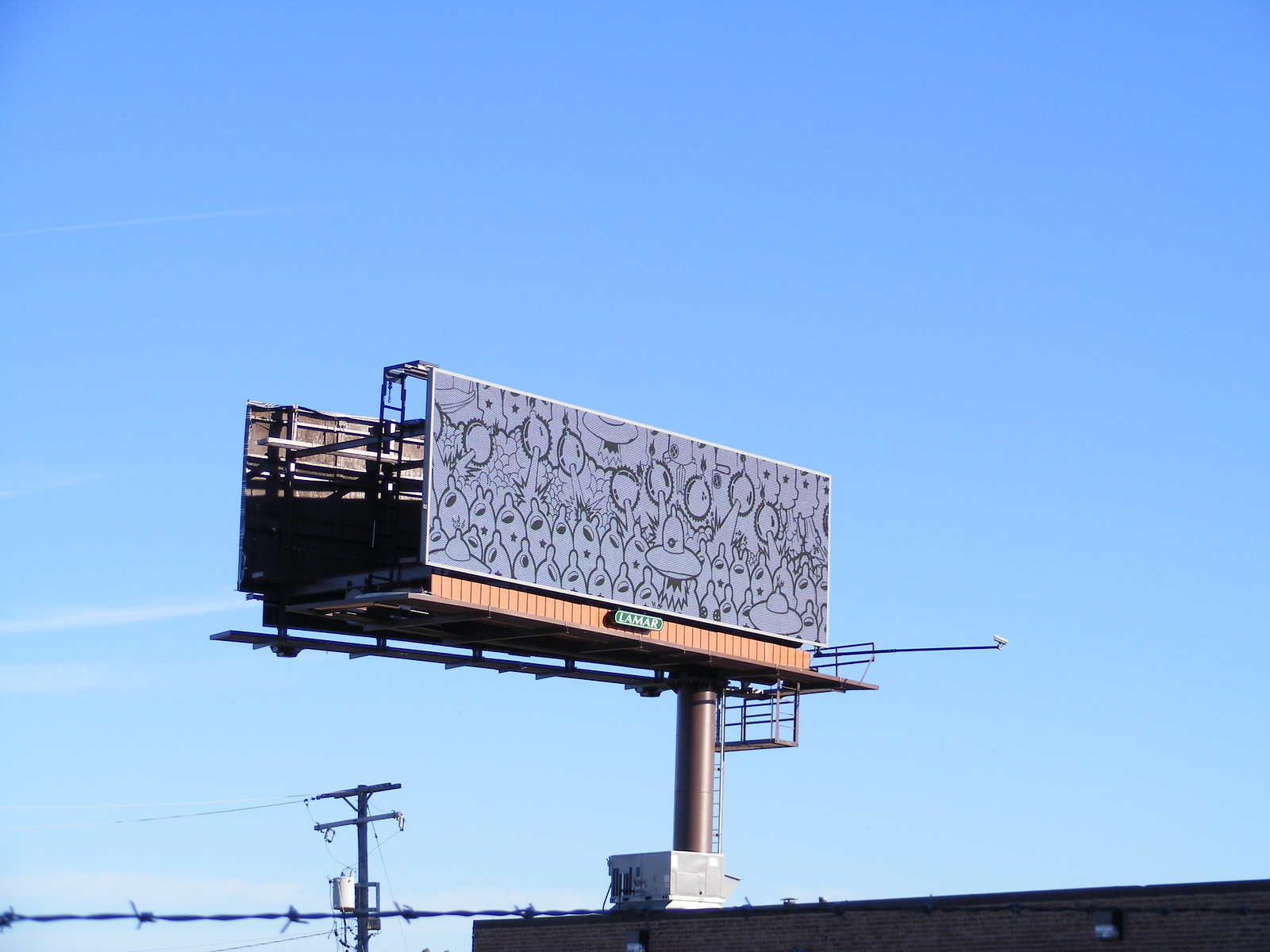A stunning color photograph captures a serene outdoor scene dominated by a clear blue sky. The gradient of the sky transitions gracefully from a richer, deeper blue at the top to a lighter hue near the horizon, hinting at the vast expanse above. Central to the scene is a roadside billboard, typical of those seen along highways. The billboard structure features a cylindrical support pillar that elevates it high into the sky. The visible billboard has no current advertisement, displaying only a random design, with the recognizable "Lamar" logo in green and white positioned discreetly underneath.

The billboard platform includes a network of rods and walking platforms at its base, hinting at the maintenance access points. A solitary link of a chain-link fence runs horizontally across the bottom edge of the image.

To the left of the billboard’s support pillar, a telephone pole stands at the lower edge of the frame, its wires extending outward and away. On the mid to lower right of the scene, the very top of a building peeks into view, where an air conditioning unit is perched, just visible in the scene. The composition captures a moment of everyday infrastructure against the endless expanse of sky.